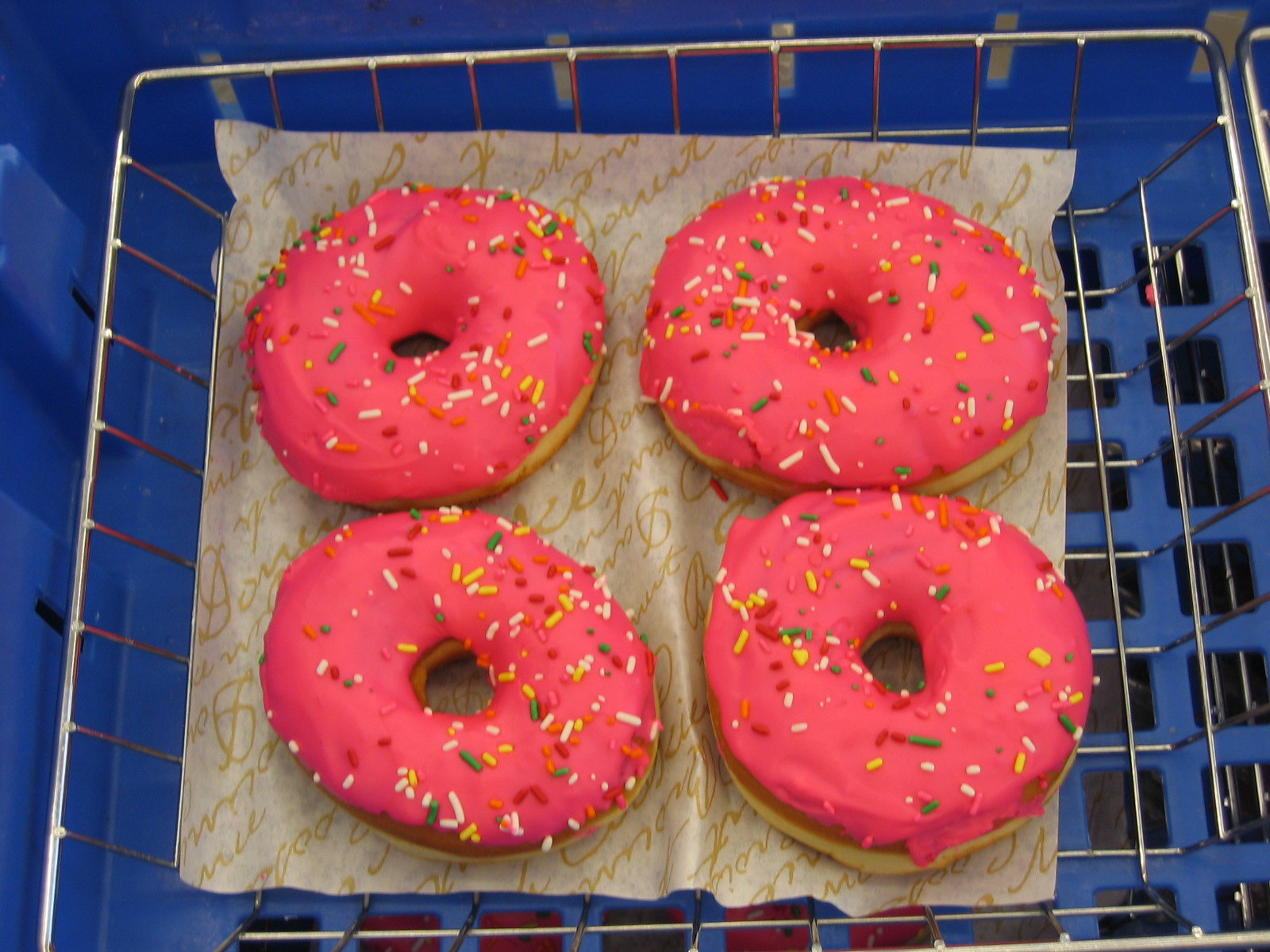In this detailed image, a top-down view reveals four donuts arranged in a square formation. These donuts have a vivid pink frosting that covers their tops and upper sides, leaving the bottom part visibly plain and light yellow. The frosting is adorned with a colorful variety of oblong sprinkles in green, yellow, red, blue, white, and orange. These delightful treats sit closely together on a piece of parchment-like paper, tan in color, featuring cursive writing that is hard to decipher. This decorative paper rests on a silver metal wire basket, characterized by its open square holes. The metal basket, in turn, is placed inside a dark blue plastic container with larger square holes on the bottom and narrow slits along the sides. The entire setup gives a visually appealing and vibrant presentation, perfect for attracting anyone with a sweet tooth.